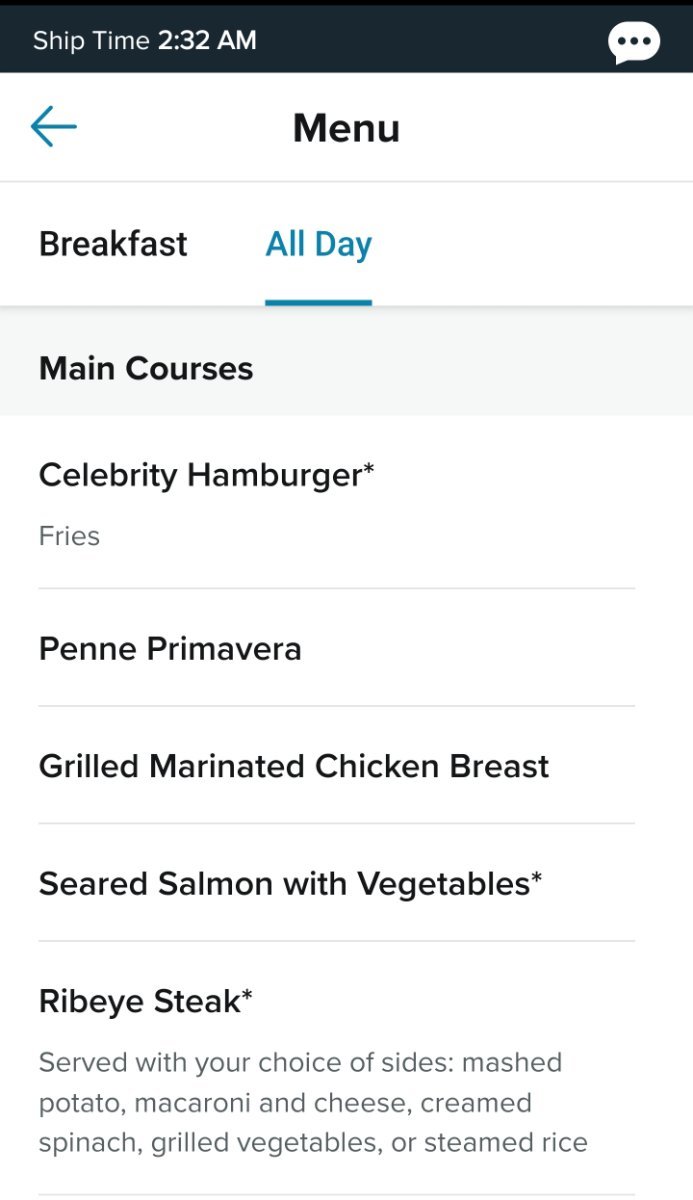This screenshot from a cell phone appears to be from a food delivery app interface. The image is portrait-oriented and it seamlessly blends with the white background, making the contents stand out.

At the very top of the screen, there is a black rectangular banner with the text "Ship Time" displayed in white. Below this title, the text "2:32 AM" appears in bold font, indicating the current time. On the upper right corner of this banner, there is a small thought bubble icon containing three dots, suggesting additional options or a menu.

Just below this top section, there is a navigation menu. On the top-left corner, a blue arrow pointing to the left is visible, likely serving as a back button. The menu shows a selection between "Breakfast" and "All Day," with "All Day" highlighted in turquoise font, indicating that it is currently selected.

The main content area of the image contains a list of menu items under the heading "Main Courses," which is displayed in a gray rectangle. The available dishes are as follows:
- Celebrity Hamburger (with an asterisk)
- Fries
- Penne Primavera
- Grilled Marinated Chicken Breast
- Seared Salmon with Vegetables
- Seared Steak (with an asterisk)

Below the listing for "Seared Steak," there is additional information in light gray text, stating "served with your choice of sides: mashed potato, macaroni and cheese, creamed spinach, grilled vegetables, or steamed rice." This indicates that the fries mentioned under the hamburger, as well as these sides, come as accompaniments to the main dishes.

The image suggests that the user is making a decision on what to order for an all-day meal, and they seem to be using a food delivery service similar to DoorDash or Uber Eats. The user is contemplating their options, weighing the choice between different entrees such as the Penne Primavera and the Celebrity Hamburger.